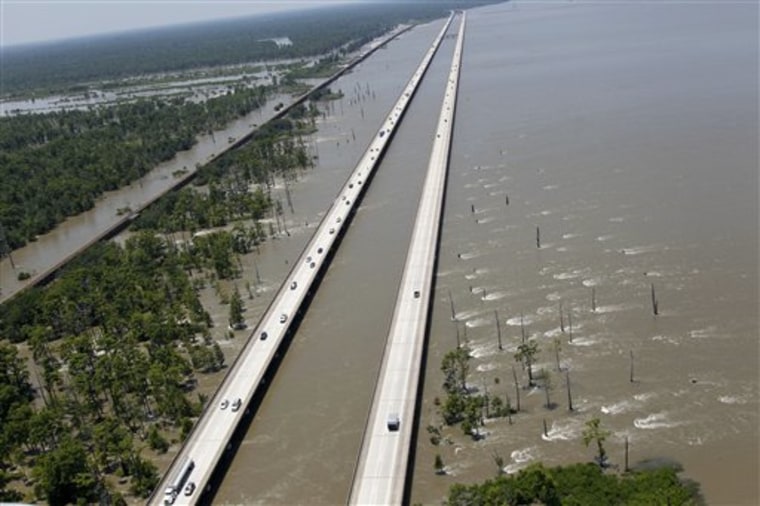This aerial photograph showcases an expansive flooded region, characterized by two exceptionally long, elevated roadways, each accommodating traffic flowing in opposite directions. These parallel roads stretch out across a vast, muddy waterway, casting a stark contrast against the submerged landscape below. On both sides of these roads, clusters of treetops poke through the water, indicating severe flooding that has engulfed the surrounding area. To the right of the roadways, the water appears to move swiftly, evidenced by visible white water sections, while on the left, denser greenery suggests a more inland position. The muddy appearance of the water, interspersed with occasional patches of blue, suggests recent flooding rather than a permanent water body. Cars, including a noticeable tractor-trailer, traverse these elevated roads, seemingly unaffected by the surrounding inundation, highlighting the unique adaptability of this infrastructure in a flood-prone environment. This scene presents a striking juxtaposition of usability amidst natural calamity, as these resilient roads continue to facilitate transportation despite the extensive flooding below.